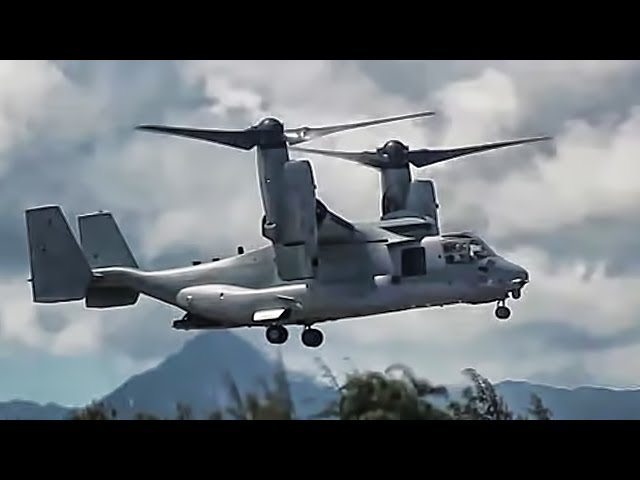The image depicts a massive, gray, military helicopter, characterized by its large rotors situated on each side of its thick body. The aircraft is hovering approximately 40 feet above the treetops, with the front and rear landing wheels extended, indicating it is near landing. The helicopter features a distinctive tail with vertical stabilizers on either side and a cockpit where a pilot is visible through the windshield. The backdrop consists of an overcast sky filled with light clouds, with mountain peaks, including a notably pyramid-shaped one, in the distance. The scene lacks vibrant colors, dominated by gray tones from the mountains and everything blending smoothly with the overcast atmosphere, though traces of green from the trees below add some contrast.